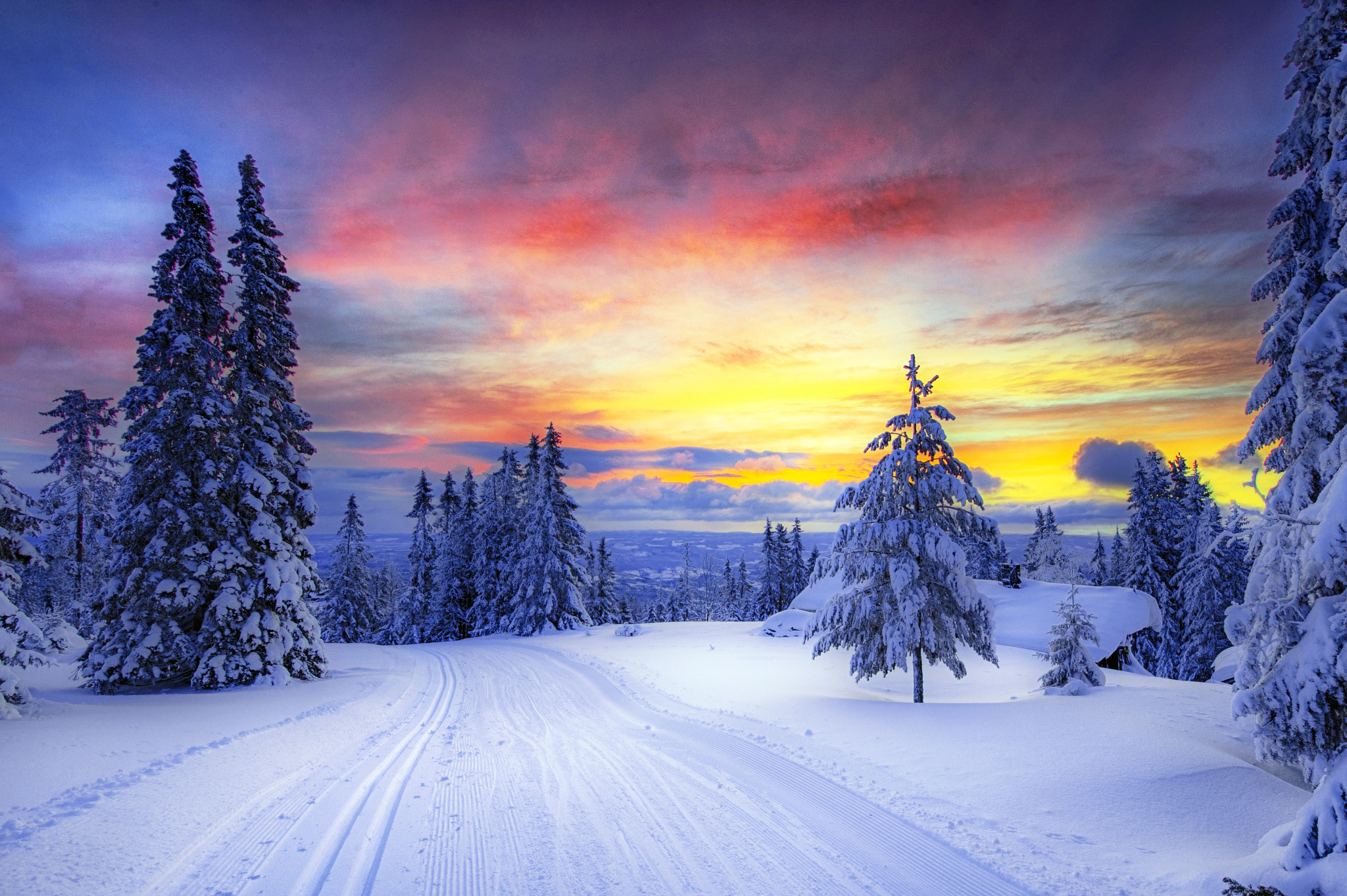This stunning photograph captures a serene winter landscape at either sunset or sunrise. The scene is set on a snow-covered trail or roadway, with visible tire tracks suggesting recent activity. Tall pine trees, dusted with snow, stand on both sides of the path, adding to the tranquil environment. In the middle right of the image, the snow-covered roof of a house peeks through the trees. The background showcases majestic mountains in the far distance, accentuating the depth and grand scale of the setting. The sky, dominating the top half of the image, is a breathtaking canvas of colors—ranging from soft pinks and purples to vibrant reds, yellows, and blues—indicative of the magical twilight hour. Patches of clouds scattered across the sky add to the overall beauty of this wintery, mountainous scene.